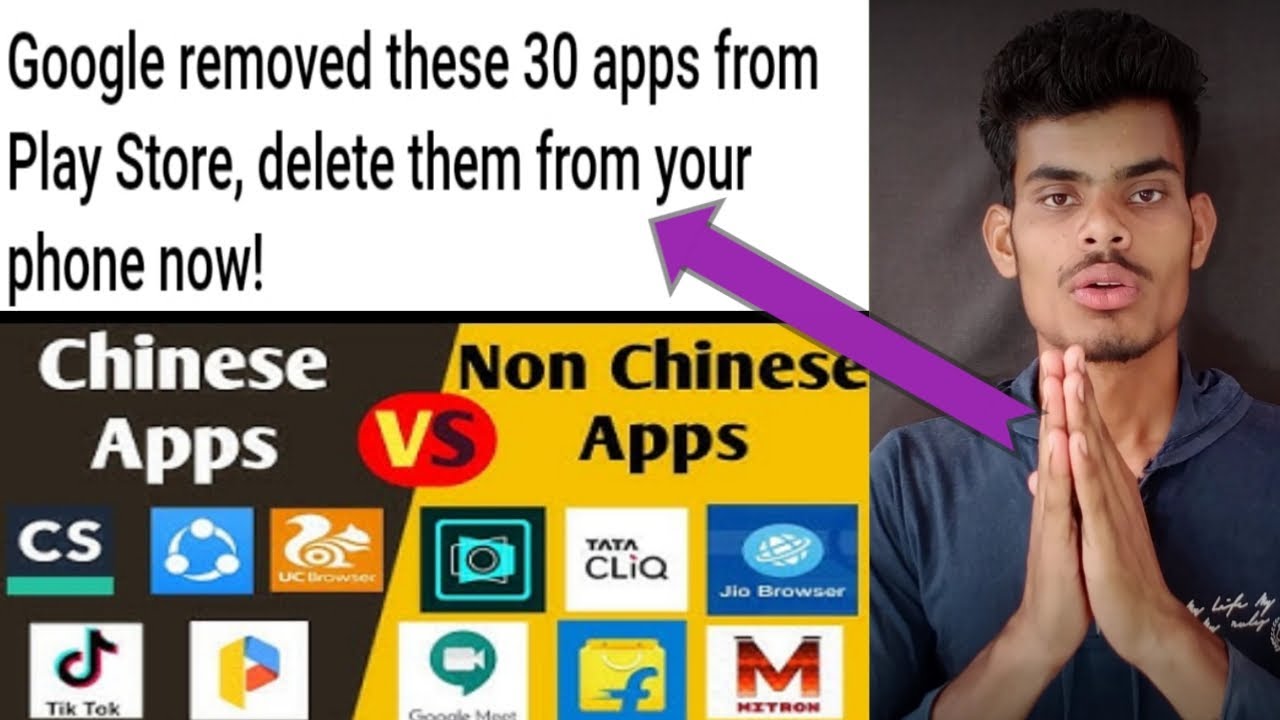The image appears to be an alarmist pop-up styled as a scammy advertisement. The main text exclaims, "Google removed these 30 apps from Play Store, delete them from your phone now!" There is a visual comparison between Chinese and non-Chinese apps.

On the Chinese apps side:
- An indistinct image with the text "Chinese apps versus non-Chinese apps."
- An icon featuring CS, depicted as a circle with three dots on a blue background.
- The UC Browser icon, represented by a white squirrel on an orange background.
- The TikTok icon.
- An app with a 'P' icon in yellow, blue, and red.

On the non-Chinese apps side:
- An icon that resembles a photo or camera.
- TATA CLiQ is featured with its logo.
- The JIO Browser icon.
- The Google Meet icon.
- An icon that appears to be related to Facebook, showing an 'F' on a yellow shopping bag against a blue background.
- The MITRON icon, showing the text "M-I-T-R-O-N" in red on a white background.

The pop-up also showcases an image of a man who appears to be of Indian or Middle Eastern descent. He is wearing a thin navy blue hoodie with the hood down, and he has his hands tented together as he looks directly at the camera. A purple arrow points from his hands to the text warning viewers to "delete them now."

Overall, the image has a sense of urgency, attempting to persuade viewers to delete the specified apps immediately.